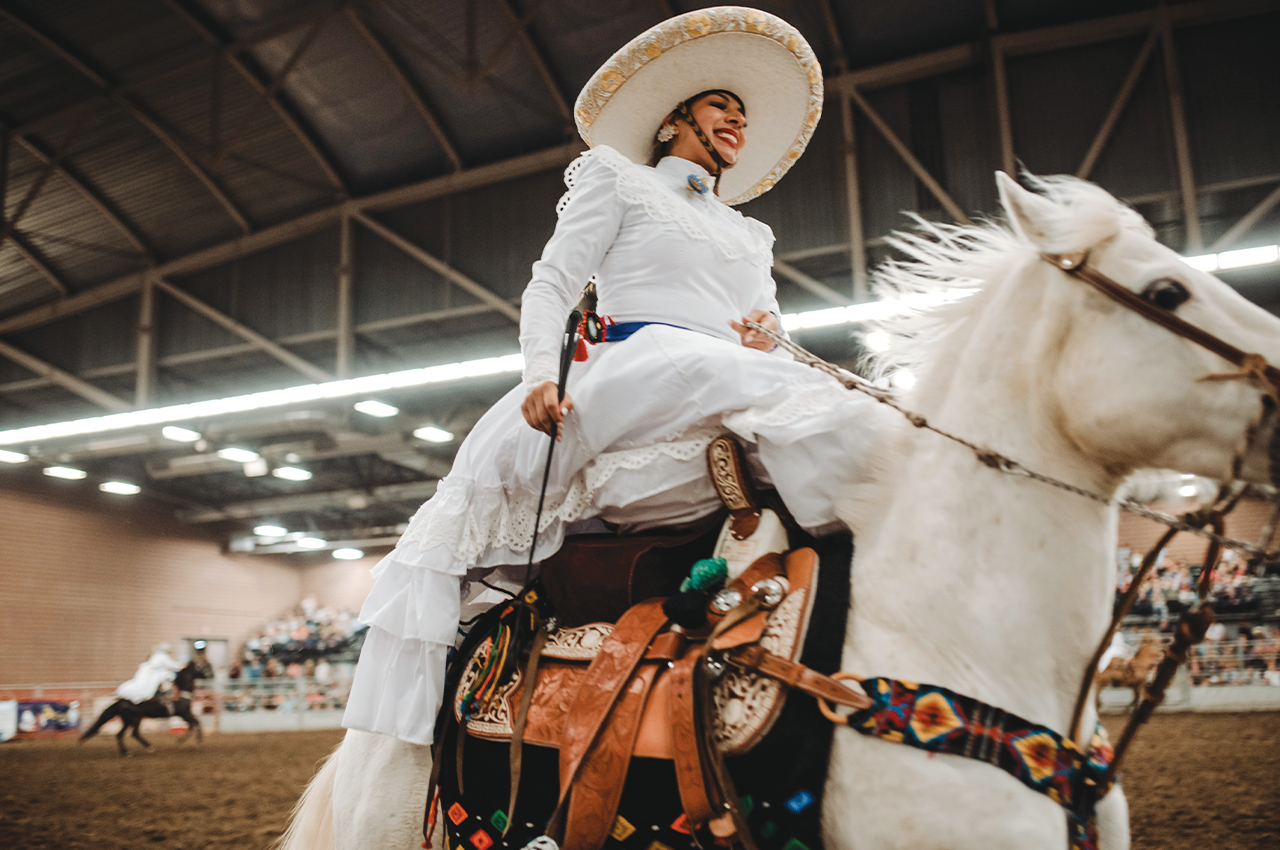A woman gracefully rides a white horse through a bustling arena, the ground beneath them a textured expanse of dirt. She wears a striking wide-brimmed sombrero, predominantly white with an intricate border of yellow and light brown, adding a vibrant frame to her face. Draped in a flowing, loose-fitting white dress that appears to brush her ankles, she exudes a sense of elegance and ease. The horse, equally magnificent, is adorned with a multicolored chest strap featuring hues of black, red, yellow, and blue. This strap secures a dark-colored bag decorated with multicolored patterns in yellow, green, and a touch of orange, complemented by brown leather straps. In the background, another woman, similarly dressed, rides a dark horse, both participants framed by the distant stands filled with captivated spectators.